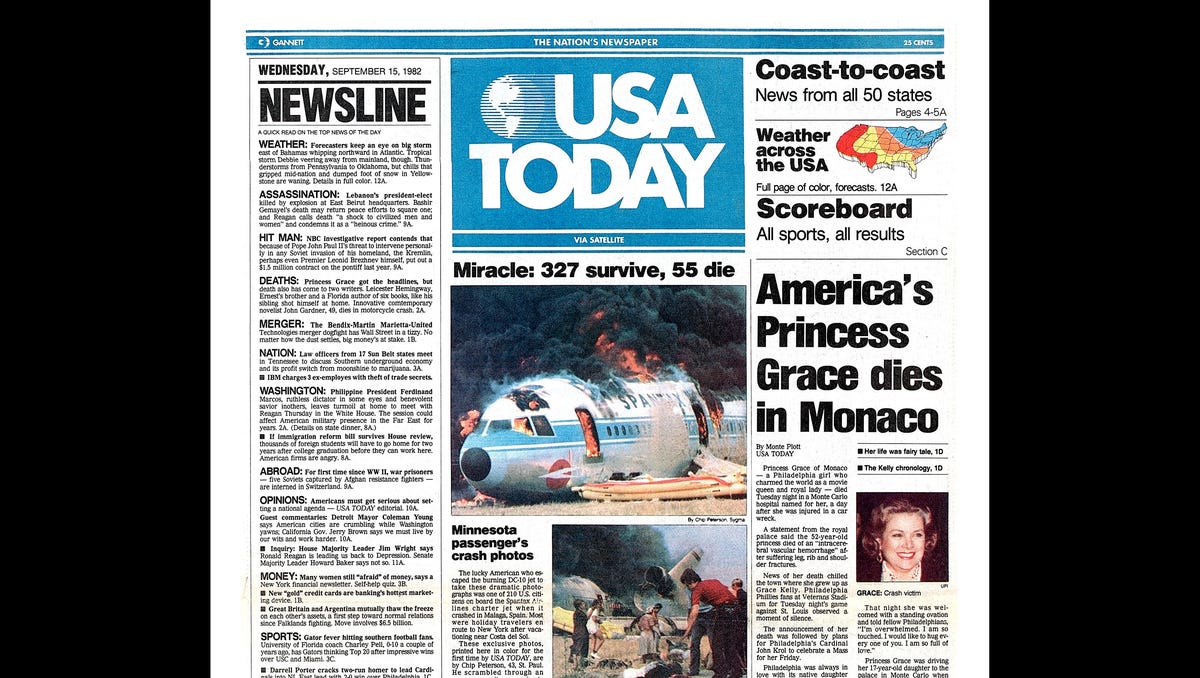This detailed image features the front page of a USA Today newspaper dated Wednesday, September 15, 1982. Dominating the page is a dramatic headline against a black backdrop with bold white text reading "Miracle: 327 Survive, 55 Die," accompanied by an image of a crashed plane ablaze on the ground. Below the headline, there is a reference to "Minnesota passengers crash photos," hinting at images and possibly stories related to the incident. A muted photograph next to this text shows various individuals, possibly workers assisting survivors. The left side of the newspaper prominently displays the "Newsline" section featuring subheadings such as Weather, Assassination, Hitman, Deaths, Merger, Nation, Washington, Abroad, Opinions, Money, and Sports, each with a brief unreadable paragraph. To the right, the section labeled "Coast to Coast" provides news from all 50 states, weather across the USA visualized with a multicolored map, and a "Scoreboard" detailing sports results. Additionally, there is a notable article headline, "America's Princess Grace Dies in Monaco," with an accompanying photo of Princess Grace Kelly, although the detailed text remains unclear.